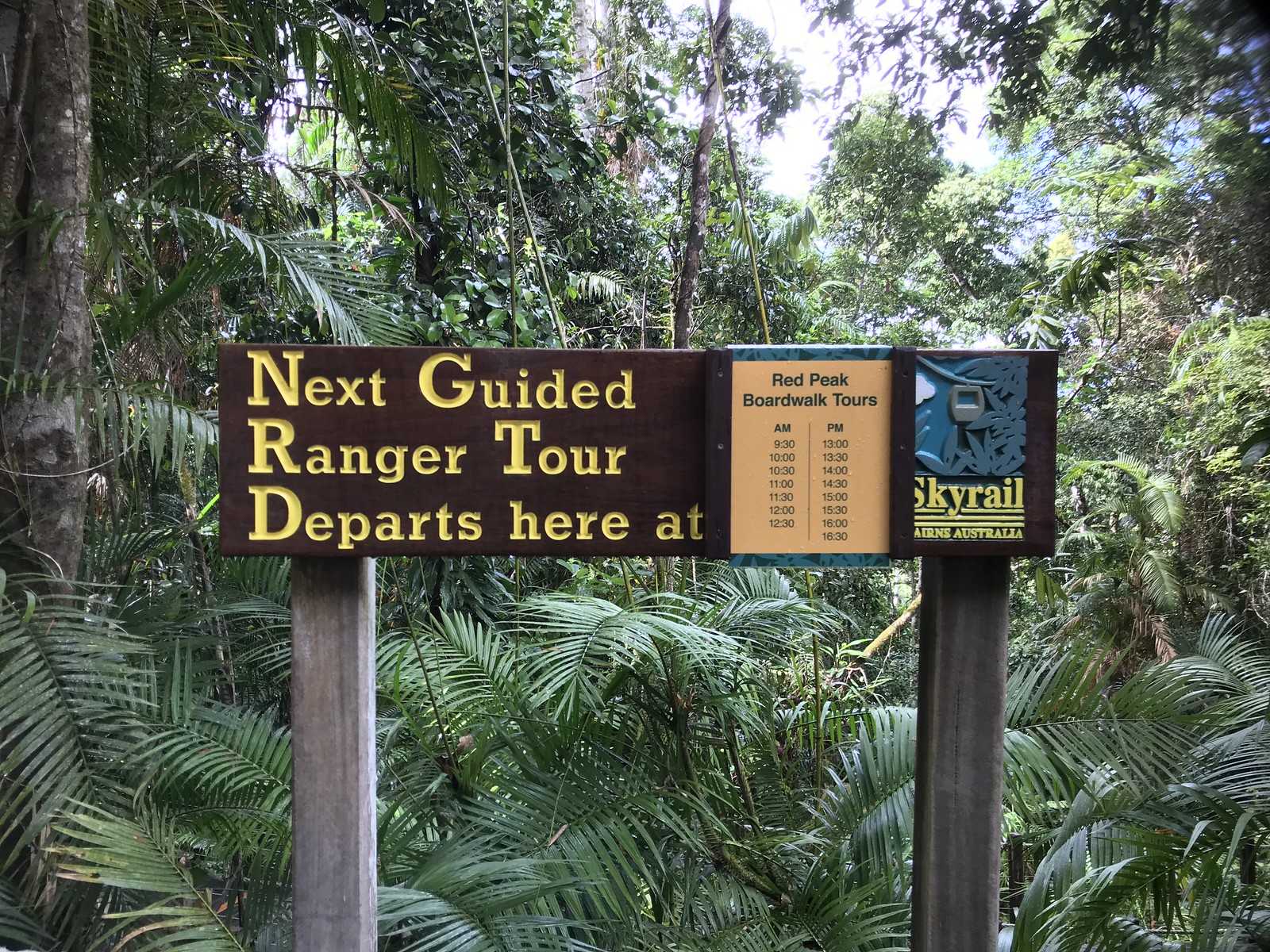In this lush, verdant scene reminiscent of a tropical jungle, a wooden sign on two sturdy wooden posts stands prominently in the foreground, surrounded by a variety of green foliage. The ground is populated by plants with long, thin blade-like leaves that split down the middle, while the left side of the image features a tree trunk devoid of branches. Centered in the background, there's a thin tree trunk or a fallen branch, partially obscured by dense, wide-blade leaves covering a fallen log. To the right, a cluster of thin, congested plants adds to the natural density of the scene. 

The wooden sign, rectangular in shape, features engraved yellow lettering that reads, "Next guided ranger tour departs here at." Attached to the right, there's a smaller glass-encased red sign detailing the "Red Peak Boardwalk Tours" schedule, listing tour departure times from 9:30 AM to 12:30 PM and from 13:00 to 16:30. Below this information, another section of the sign displays a carved emblem of a Skyrail system and the inscription, "Skyrail Cairns Australia." Bathed in natural sunlight filtering through the trees, the vibrant greenery suggests a sunny summer day, enhancing the sense of a thriving, tropical wilderness.